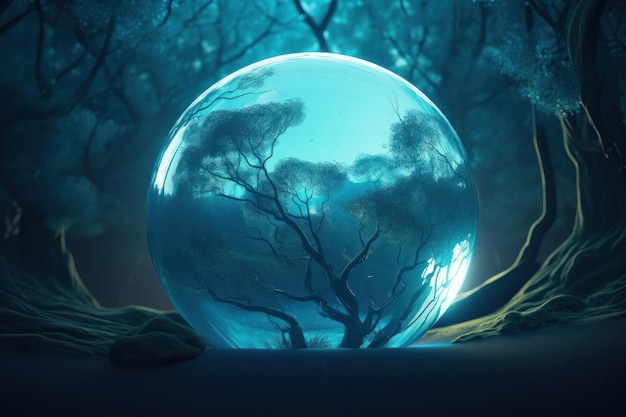Set against a dark and eerie forest background, this detailed illustration features an enigmatic crystal ball resting on the ground. The forest is shadowy and somber, with brown trunks and almost blackish-green leaves that seem to wither under the dim light. At the center of this horizontally aligned image, the crystal ball stands out, emitting a ghostly blue hue that spills over its surroundings. Inside the crystal ball, a seemingly otherworldly scene unfolds: the top portion of an ancient, nearly dead tree whose gnarled branches are largely leafless, save for a few struggling leaves at the top. The ball also reflects the sky above, adding pockets of a lighter, bluish color to the internal scene. Encircling the crystal ball are more trees and branches from the forest, appearing distorted and curvaceous outside the mystical sphere. The interplay of light and shadow, along with the transparent, glassy surface of the ball, creates an ethereal atmosphere that blurs the lines between night and day, reality and another realm.